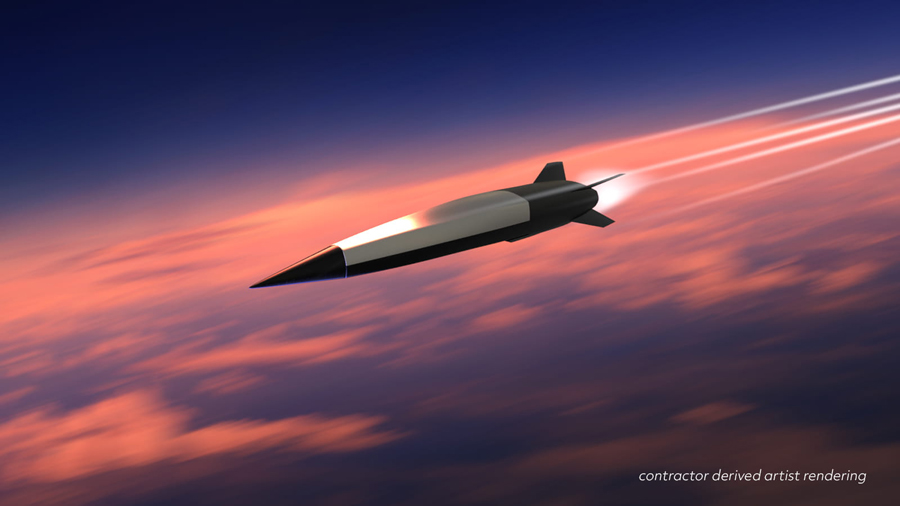The image depicts a computer-generated or artist-rendered scene, prominently featuring a sleek rocket or missile piercing through a vibrant sky. The sky is a deep, dark blue, accentuated with clouds in striking hues of pink, orange, purple, and dark blue. The rocket, central to the image, has a distinctive black pointed tip and base, a white or gray body, and a black underside. Behind the rocket, fiery exhaust and trailing white smoke illustrate its fast movement from right to left, suggesting a high-speed flight. The bottom right-hand corner of the image contains the text "contractor derived artist rendering," confirming the image's origin.